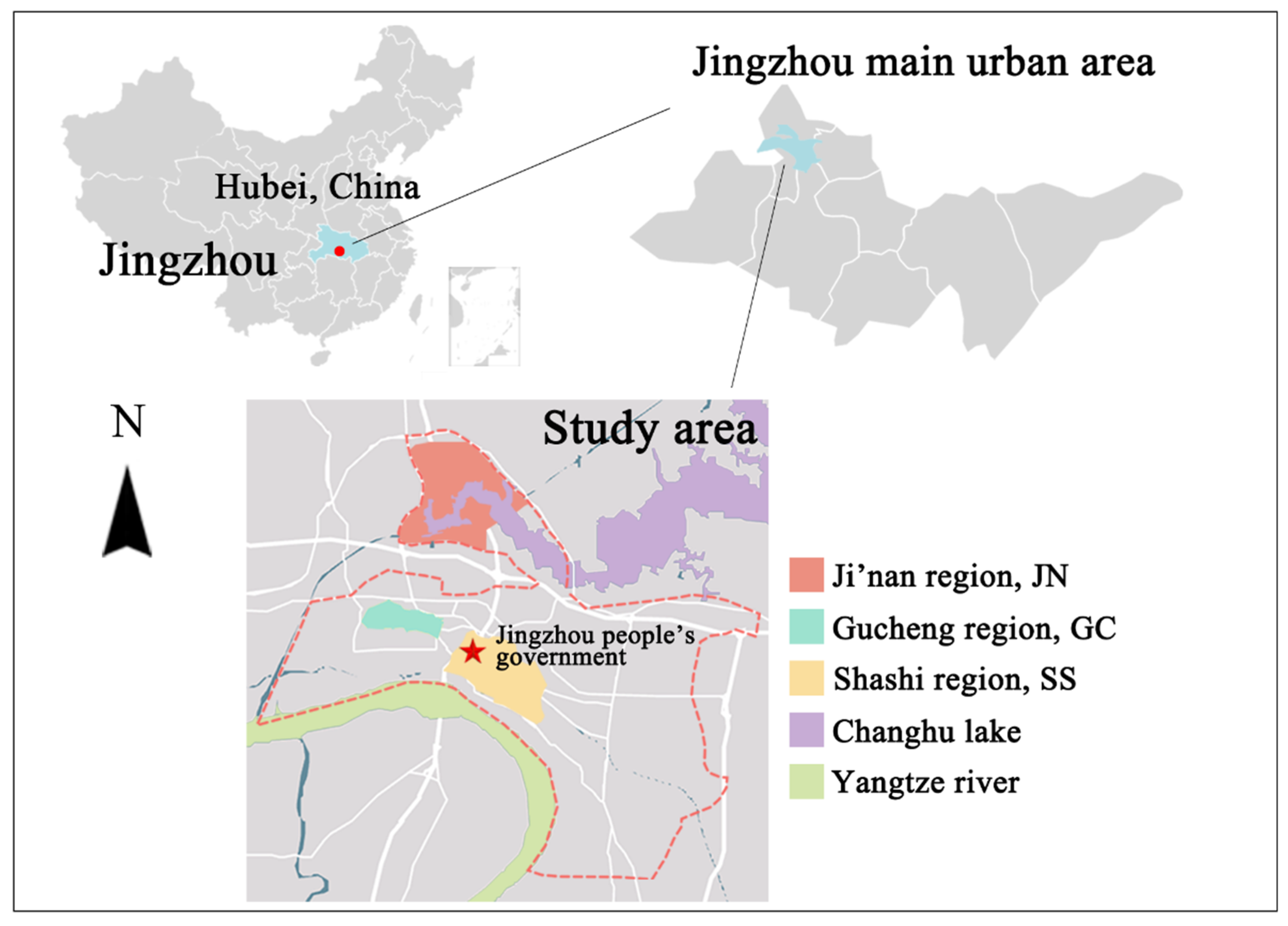The image is a detailed infographic focusing on the Jingzhou region in Hubei, China. In the top left corner, it features a map of China with the Hubei province highlighted, specifically pinpointing Jingzhou. The top right corner presents a zoomed-in view of the Jingzhou main urban area, labeled clearly. Below, there is a further magnified section displaying the study area within Jingzhou. This section highlights several regions and geographical features, each marked in distinct colors: the Jinan region in red, the Gucheng region in blue, the Shaxi region in yellow, the Chengdu Lake in purple, and the Yangtze River in green. A key to the right of the map explains these color codes, ensuring each area is easily identifiable. The map and its elements are set against a white background, with the primary map in a gray silhouette, providing clear visual contrast.